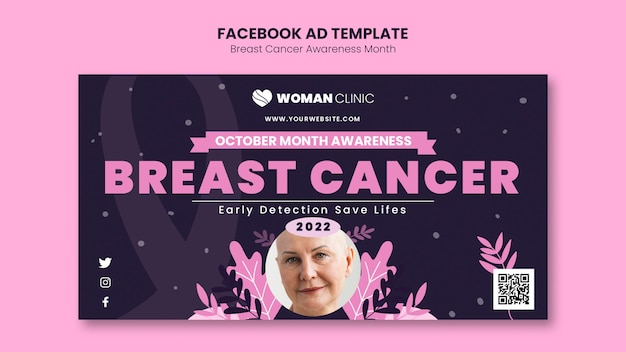This image features a webpage or sign with a pink background, prominently highlighting Breast Cancer Awareness Month. At the very top, a header reads "Facebook Ad Template," with "Breast Cancer Awareness Month" written just below.

The center of the image is dominated by a black box, accented with small gray dots, and featuring the silhouette of a pink ribbon symbolizing breast cancer awareness. The name "Women Clinic" is displayed at the top of this box, along with the URL "www.yourwebsite.com."

A pink banner stretches across the middle of the black box, bearing the message "October Month Awareness" in white letters. Centrally placed below the banner, bold text reads "Breast Cancer," followed by a white line and the crucial message "Early Detection Saves Lives."

The image features a woman without hair, likely indicating her battle with cancer. She has a slight, stoic smile on her face, capturing a moment of resilience. The year "2022" is denoted next to her.

Social media icons for Twitter, Instagram, and Facebook are situated in the lower-left corner, while a scanning area is placed in the lower-right corner of the image.